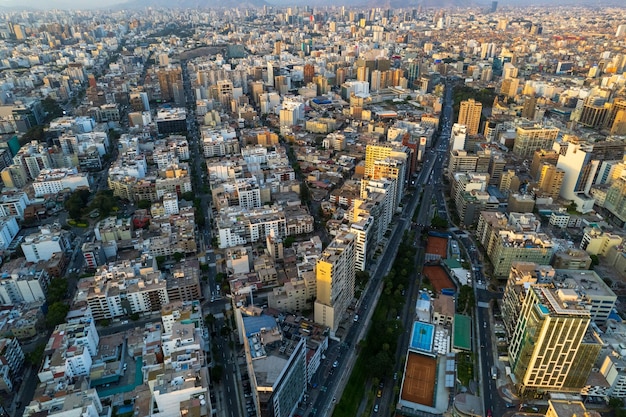An aerial photograph captures a sprawling, densely populated cityscape, teeming with tall buildings that stretch endlessly to the horizon, where a faint haze or possible pollution grays the skyline. The city is a labyrinth of architecture, with buildings densely packed together, resembling dots and forming an intricate urban patchwork. At the lower portion of the image, the structures converge into a V-shaped pattern, with streets threading between them. Prominent thoroughfares cut through the city, one veering towards the top right and another slightly left of center. Toward the right, rows of smaller, brown rooftop structures, possibly apartments or stores, break the monotony of high-rise buildings. An assortment of orange and blue crates is also visible in this area, adding a splash of color amidst the rigid grid of buildings. The sun casts light upon the left side, illuminating the tops of the countless buildings that dominate the image.